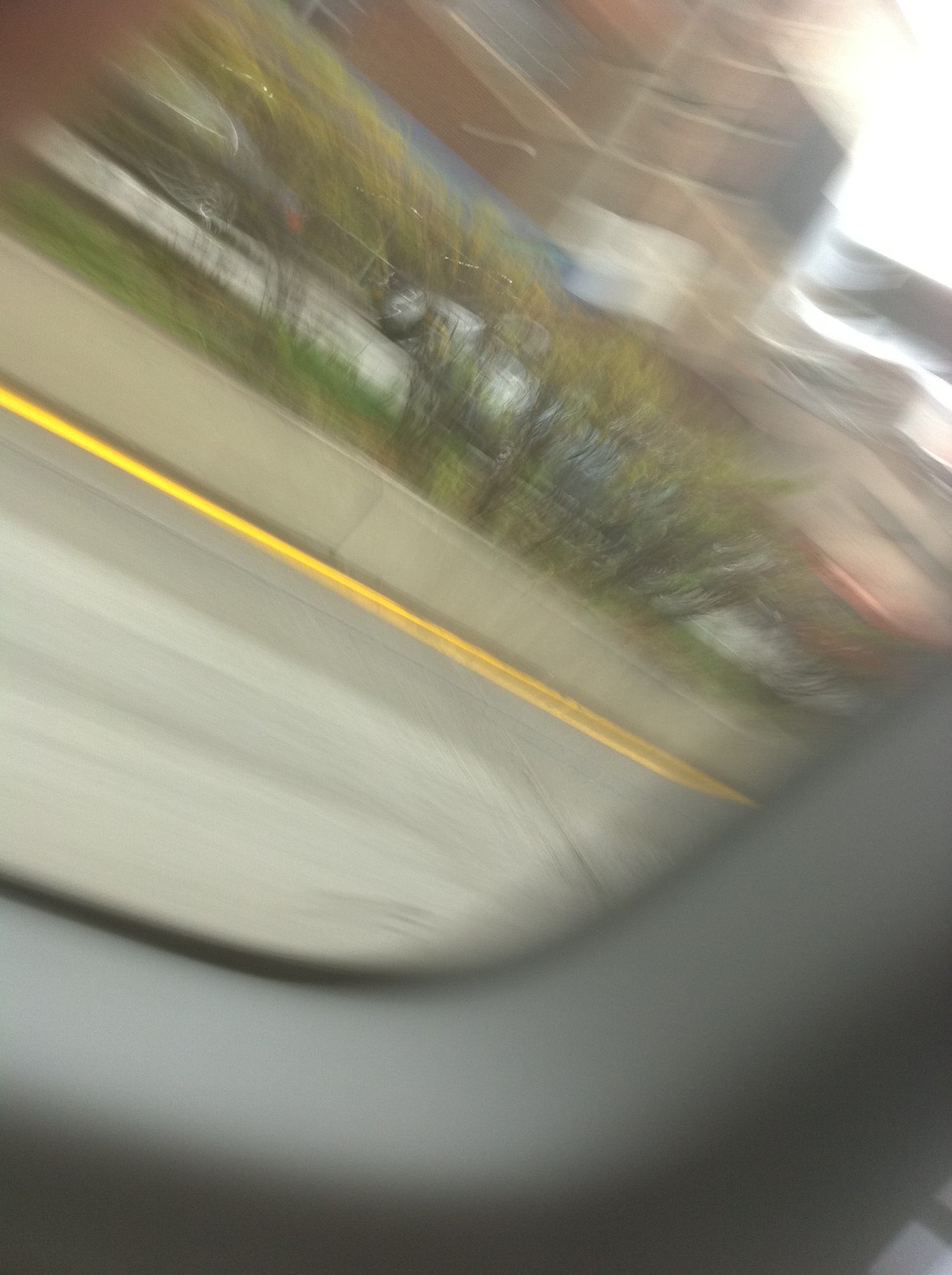The photograph appears to have been taken from within a moving vehicle, possibly a van or a car, as indicated by the visible motion blur. In the bottom right corner, the edge of a dark grey window with a slight curve is noticeable. The grey road below features a yellow line near its edge, leading to a small concrete ledge. Beyond the ledge, green bushes provide a burst of color before giving way to a red building in the background. The top right corner of the image reveals a glimpse of a white sky, adding to the overall sense of motion and depth in the scene.